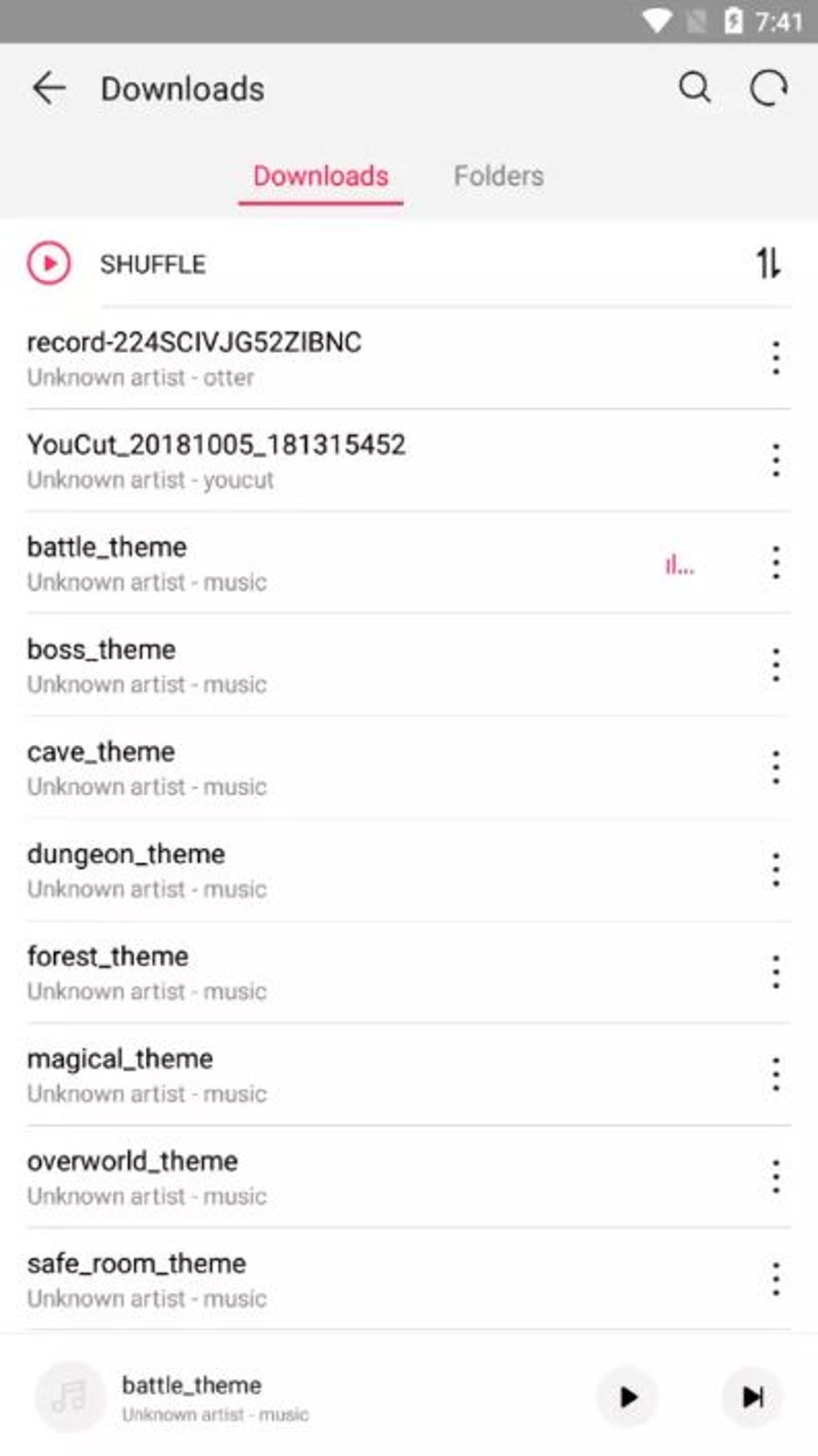This is a detailed description of a screenshot from a smartphone displaying a downloads list, predominantly consisting of music files. At the very top of the image, there is a dark gray status bar, below which lies a lighter gray navigation bar. In the upper left-hand corner of this lighter gray bar, "Downloads" is written next to a back arrow. Underneath, another line reads "Downloads," highlighted in red and underlined; next to it, the word "Folders" appears but is grayed out.

Below this section is a row featuring shuffle controls, marked by a red circular button with a white shuffle icon inside it. Following this are 11 entries of downloadable music files, each with a title and "Unknown Artist" listed as the creator. The songs are titled as follows:

1. Record (followed by a string of numbers and letters) - Unknown Artist
2. You Cut (followed by a string of numbers) - Unknown Artist
3. Battle_theme - Unknown Artist, Music
4. Boss_theme - Unknown Artist, Music
5. Cave_theme - Unknown Artist, Music
6. Dungeon_theme - Unknown Artist, Music
7. Forest_theme - Unknown Artist, Music
8. Magical_theme - Unknown Artist, Music
9. Overworld_theme - Unknown Artist, Music
10. Safe_room_theme - Unknown Artist, Music

To the right of each music entry, there are three vertical dots, presumably for accessing additional options or actions related to each file. At the bottom of the screen, the currently playing song is "Battle_theme," which is indicated by a small music player interface displaying the track.